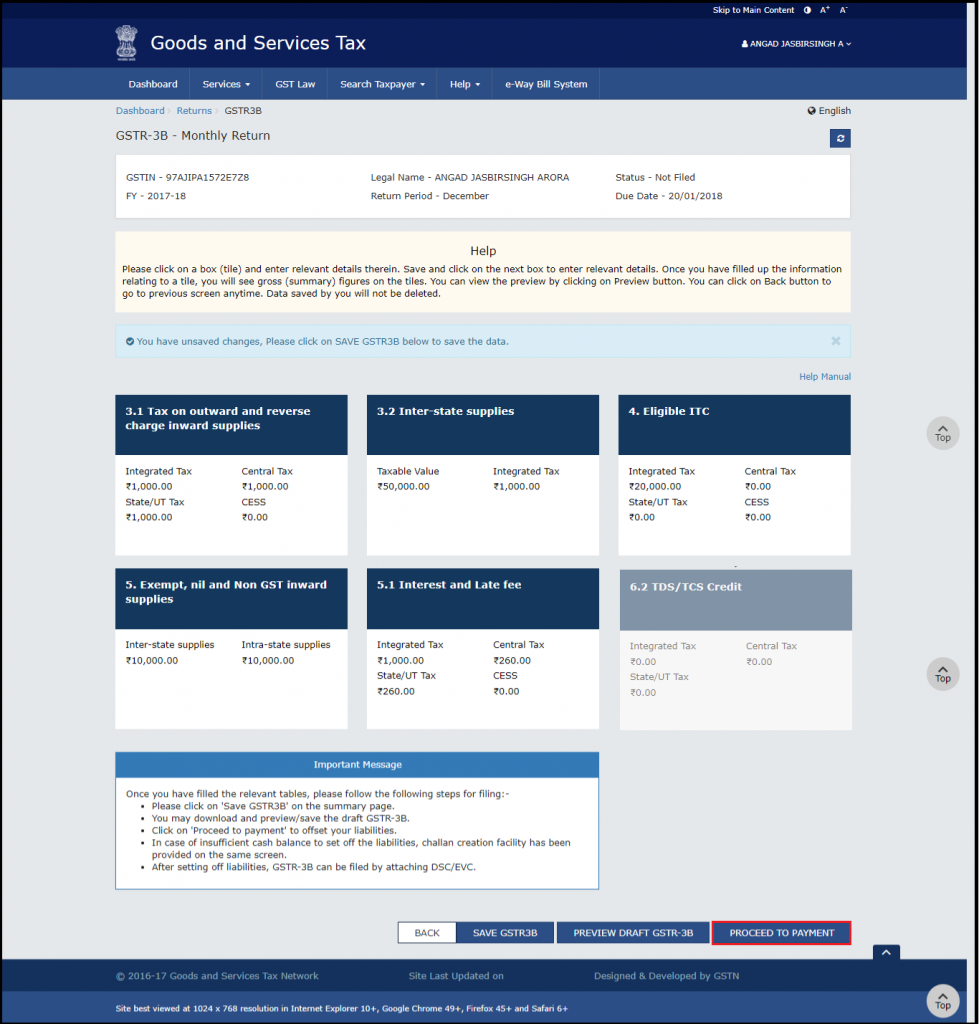This screenshot captures the interface of a British government website dedicated to goods and services tax management. The header is a dark blue banner prominently featuring a crown icon on the top left corner, followed by the text "Goods and Services Tax" in white font. Adjacent to this, on the far right side of the header, is a small white login icon accompanied by a user's name.

Directly beneath the main header is a thinner, lighter blue navigation bar. This bar contains a row of interactive categories: Dashboard, Services, Search, Help, and ePay File.

The body of the website starts with a gray section in the top left corner displaying a code and the phrase "Monthly Return" in a monospace typeface. Below this, the content area is divided into several distinct sections. A large white box at the top lists "Numbers, Name, Return Period, Status, and Due Date."

Following this, a sizable tan box labeled "Help" is centered with a helpful tip underneath. Further down, a very thin green box containing a checkmark icon indicates the presence of unpaid charges, along with a prompt to "Click on 'Save' to save the data." 

Toward the middle, there are six square boxes arranged in a 2x3 grid format, each detailing different fee schedules and percentages to pay. Additionally, a larger white box near the bottom highlights an "Important Message" within a blue banner.

At the very bottom right section of the page, there are navigational buttons: "Back," "Save," "Preview Draft," and "Proceed to Payment." Notably, the "Proceed to Payment" button is accentuated with a red outline to draw attention.